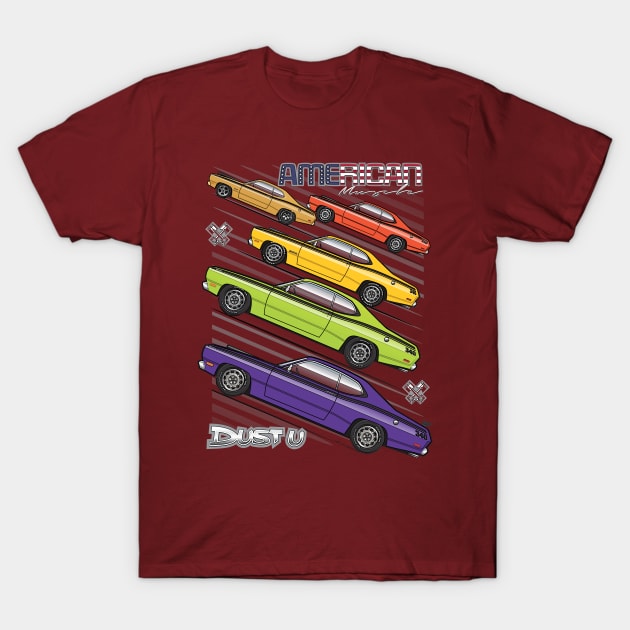This is an illustration of a maroon red t-shirt on a flat white background. Prominently featured on the t-shirt are five muscle cars, each ascending diagonally to the left at approximately 30 degrees. The largest car at the bottom is purple, with progressively smaller cars above it: a lime green car, a mustard yellow car, and a pair of smaller cars at the top—a dark gold yellow car on the left and a bright red car on the right. Above these cars, the word "American" is displayed, with "A-M-E" in blue adorned with white stars and "R-I-C-A-N" in red and white stripes, mimicking the American flag. Beneath this text, there is some indecipherable cursive writing. Flanking the yellow car to its left and the purple car to its right are sets of crossed metallic spades. The entire car arrangement is set against background stripes of gray, angled similarly to the cars. At the bottom, under the purple car, there is graffiti-style text in shiny black and white that reads "Dust U."